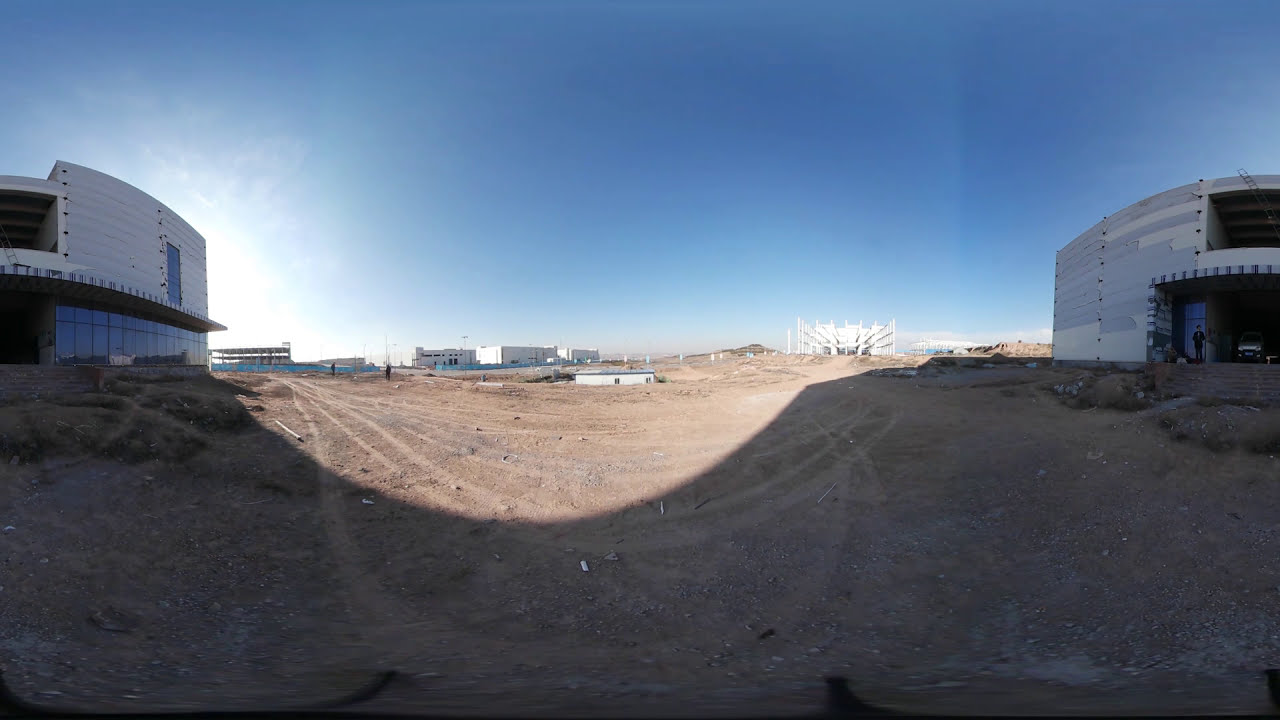The image showcases a construction site prominently featuring a low, central warehouse building surrounded by a dirt lot marked with tire tracks. On either side of the image are partially visible unfinished buildings with large open frames, suggesting ongoing construction. The scene is set under a clear blue sky with no clouds, typical of midday lighting. To the left, a sunflower and sun flare are present, along with possible artifacts from a dirty lens, while the lower half of the image is shaded, likely from an unseen building. The colors visible include various shades of blue, white, gray, green, tan, and silver, contributing to the scene’s industrial and outdoor daytime setting. The image might be slightly warped, indicative of a 360-degree camera effect, giving an illusion of the buildings wrapping around the scene.